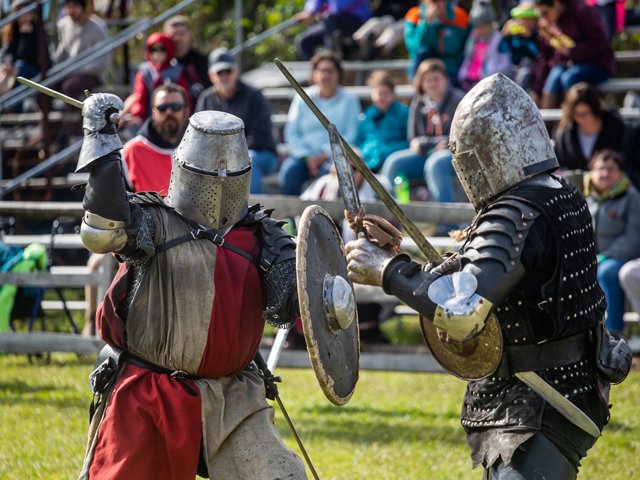In the photo, two gentlemen are engaged in a medieval knight reenactment outdoors. The scene features a set of bleachers behind a fence line, filled with spectators dressed in modern-day clothing, watching the duel.

The knight on the left is outfitted in red and white attire with chainmail sleeves and arm armor. He wears a silver bucket helmet with eye slits and pinholes for ventilation. His gear includes a round shield on his left arm, metal gloves, and a belt carrying swords. He is actively swinging his sword overhead with his right hand, preparing for an attack.

Opposite him, the knight on the right is dressed predominantly in black, sporting a metal helmet, gloves, and a black leather jacket adorned with silver studs. He holds a small, lowered shield and brandishes both a knife and a sword, seemingly bracing for the incoming strike. The lighting suggests the scene takes place in the evening, with cool weather implied by some spectators wearing heavy jackets.